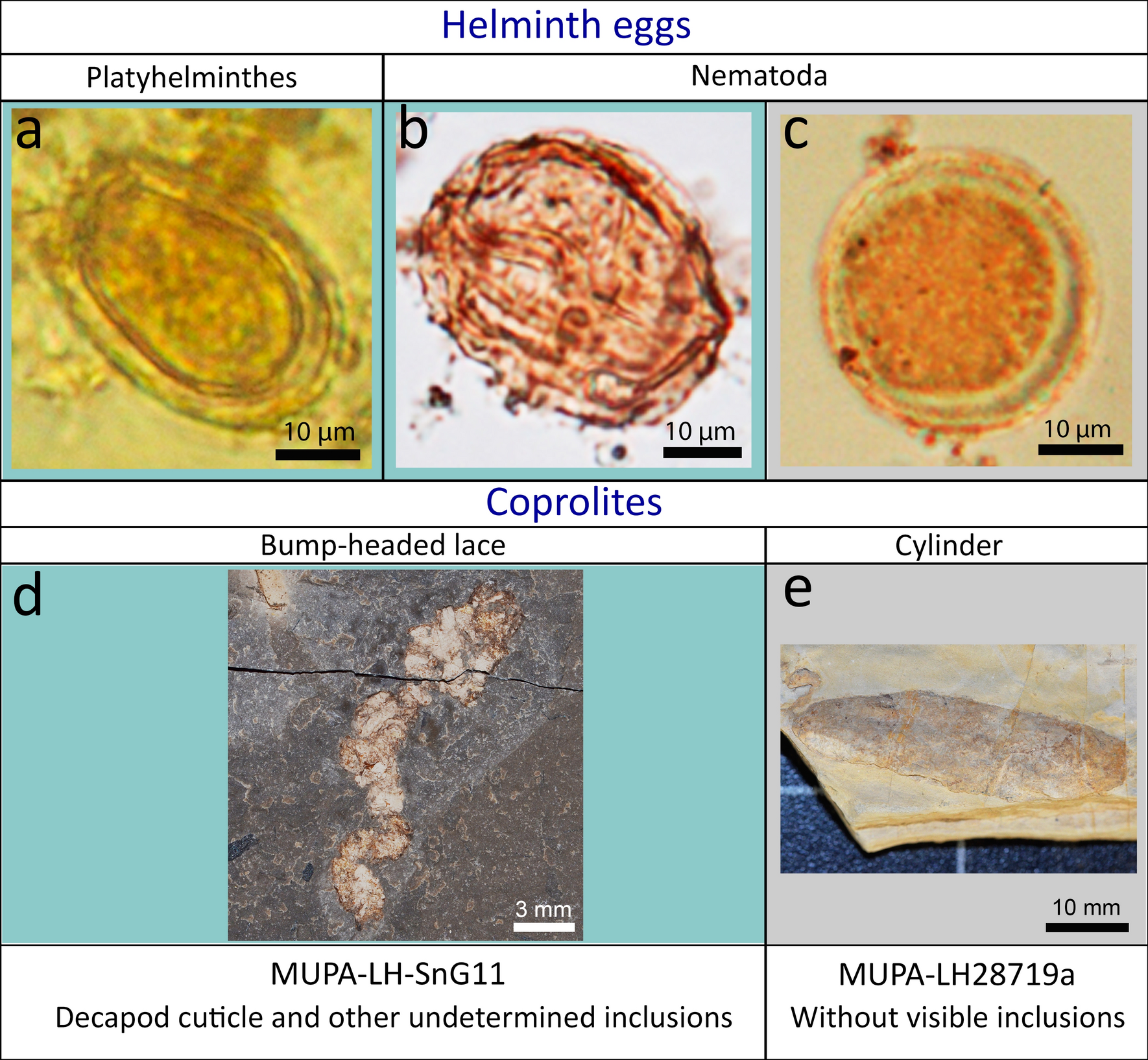The image is a rectangular chart titled "Helminth Eggs" in royal blue at the top, displaying intricate microscopic views of various helminth eggs and related structures across five labeled panels: A, B, C, D, and E. The chart is divided into three categories: "Platyhelminthes," "Nematoda," and "Coprolites."

Panel A, labeled "Platyhelminthes," depicts a cellular structure with a yellowish-golden hue, featuring a darker oval at an angle and subtle internal lines. A thick black line in the corner reads "10 μm," indicating the scale. Panel B, under the "Nematoda" category, shows another cellular organism with a white background, a pinkish-red body, and intricate internal lines, also scaled at 10 μm. Panel C, also labeled under "Nematoda," displays a more circular, orange organism with an irregular shape on a beige background, maintaining the 10 μm scale.

The lower section labeled "Coprolites" consists of two panels. Panel D, titled "bump-headed lace," presents a larger, dark gray sample with light gray inclusions and a central light beige structure resembling a thick line. This image includes a "3 mm" scale marker. Finally, Panel E, labeled "cylinder," features two grayish-tan, papyrus-like folds without visible inclusions, marked with a "10 mm" scale. Both panels include additional labels with specific identifications and descriptions.

The images vary in color, primarily featuring yellow, red, brown, and beige organelles, all detailed with subtle inner structures, emphasizing their biological nature and differing scales, ranging from 10 micrometers to 10 millimeters.